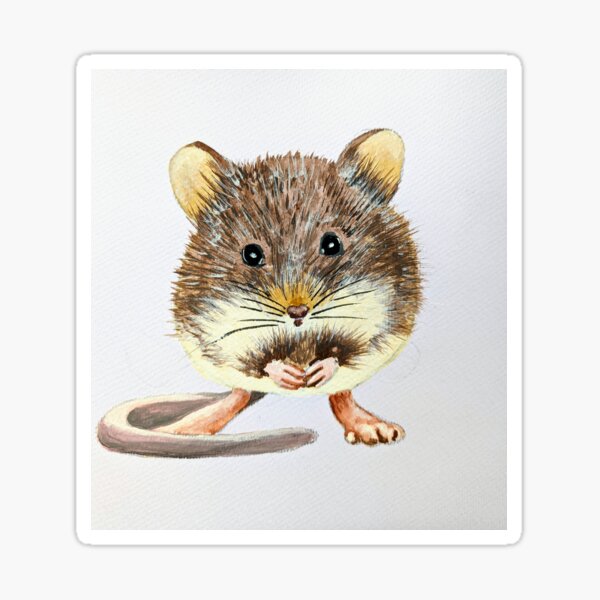This detailed image features a hand-drawn depiction of a small rodent, likely a gerbil or mouse, set against a gray square background. The image also includes a white border framing the tiny square. The creature is characterized by its round, almost circular body with a light beige chest that has a small brown spot. The rodent sits upright on its hind legs, with its two ears erect and facing forward. These ears are a chocolate brown on the outside and a lighter beige on the inside. The animal's fur exhibits tiny brown hairs, adding to its realistic texture.

The face of the rodent is adorned with two small black eyes and a tiny brown nose surrounded by delicate brown whiskers. The round mouth is visible just below, and it seems to be holding a nut or seed with its front paws, which are a rosy pinkish color. Both the hands and feet are similarly flesh-colored, and the front paws are clasped together, emphasizing the lifelike pose.

A long, slender tail, gray in color, extends from the back of the rodent and wraps around to cover one of its large feet, adding an element of depth to the drawing. The overall composition and meticulous details, such as the texture of the fur and the subtle coloration of the body parts, make this a captivating and realistic representation.